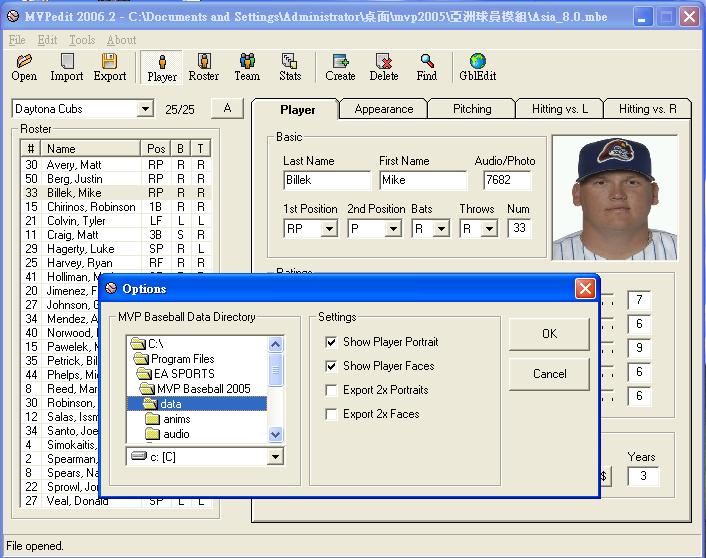The image depicts a slightly dated computer program window, likely from the 90s, with a predominant blue heading featuring white text that displays file information. Along the upper right of the window are the typical minimize, maximize, and red X buttons. The main background of the window is a tan color. At the top left, you can see recognizable menus such as File, Edit, Tools, and About.

To the right of the main window, there is a headshot of a baseball player, identified as Mike Billick, a right-handed pitcher wearing a blue cap with an insignia and a blue striped uniform. His detailed stats are displayed, noting he bats and throws right, and wears the number 33. The player menu on the left lists numerous players, around 25 or 26, indicating a roster selection.

Superimposed on this main window is a smaller "Options" sub-window with a blue header and a tan background. In the upper right of this sub-window are the minimize, maximize, and red X buttons, and it displays options such as program files, EA Sports, MVP Baseball, among others, with "OK" or "Cancel" buttons towards the bottom right. The overall setup and interface, including elements like the menu names and structure, suggest that this software governs baseball player statistics and organization.